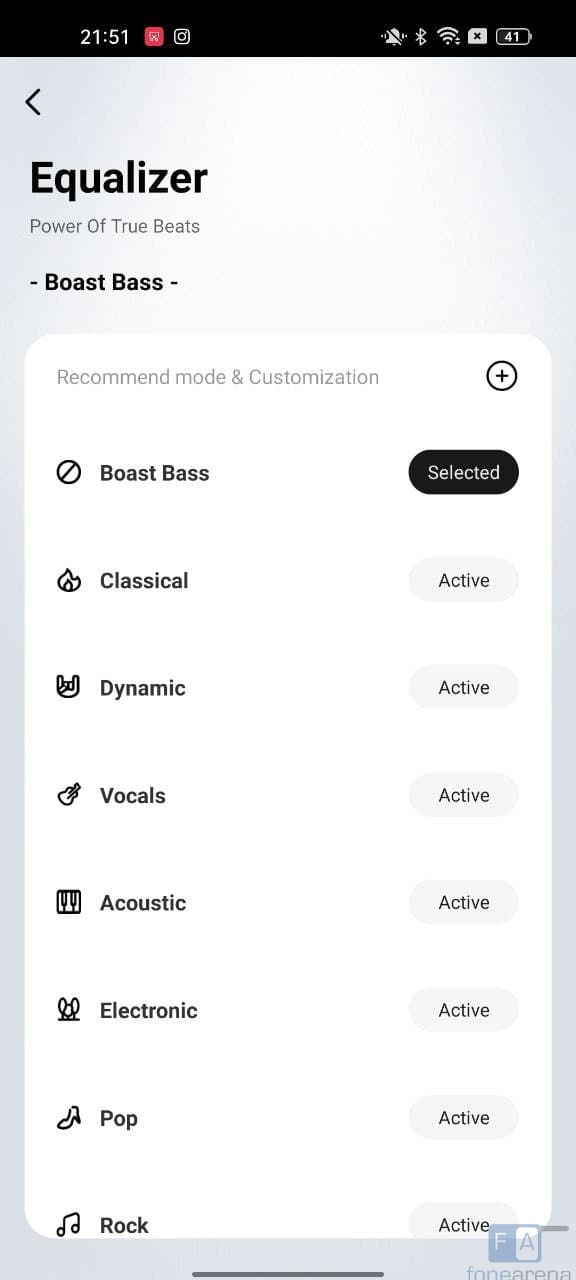Here is a cleaned-up and detailed caption based on the description provided:

---

This is a detailed screenshot from a smartphone display. At the very top, there's a black border. On the left side, an inch from the edge, the time is displayed in white as 21:51. Right next to it, there's a red square and an indistinct white icon, followed by a camera icon. On the right side, there's a battery icon displaying 41% charge in white. Next to it, a gray square contains a black 'X', followed by the Wi-Fi, Bluetooth (which is turned on), and sound (which is turned off) icons. 

Below this section, there's a blue border. In the top left corner is a greater-than sign pointing left. Underneath this, in large, bold black letters, is the word "Equalizer." Beneath that, in smaller black letters, it reads "Power of True Beats." Below this is a dash, followed by "Boast Beats" in bold, another dash, and finally a descriptive white tab that extends down to about an inch from the bottom. Along the sides and across the bottom is a light blue steel background. Across the top of this white tab, it states "Recommended Mode and Customization." 

On the left side of the tab, a white circle with a black border and a black plus sign inside is visible. Running down the left side are eight icons, each followed by a label: "Boast Bass," "Classical," "Dynamic," "Vocals," "Acoustic," "Electronic," "Pop," and "Rock" at the bottom. On the right side of this tab, there are tabs listed vertically. The top tab is black with the word "Selected" in white. Below it, subsequent tabs are gray and black, with the word "Active" written on them. In the bottom left corner of this tab, partially cut off, are the words that appear to read "for Arena."

---

This version of the caption is detailed and structured for clarity, providing a descriptive account of the screenshot's content.